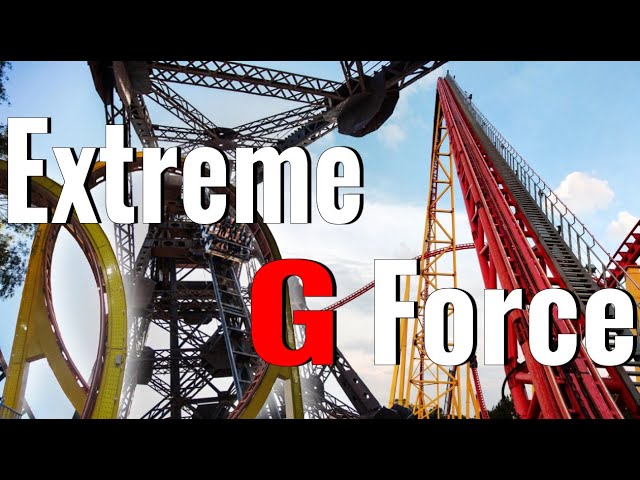The image depicts an upward view of an outdoor roller coaster scene, featuring multiple vibrant roller coasters amidst a sky filled with clouds. On the right side, a red and yellow roller coaster track appears to ascend steeply before plunging dramatically. To the left, there are black and yellow tracks, possibly part of a corkscrew-shaped roller coaster, with another black track in the middle that seems to spiral. Prominent white and red text overlays the scene, reading "Extreme G-Force." The word "Extreme" is positioned in white on the top row, outlined with a black drop shadow, while "G-Force" is displayed on the second row, with "G" in bold red text and "Force" in capitalized white letters, both also shadowed in black. The entire image is letterboxed with black rectangles on the top and bottom, adding a cinematic touch to this thrilling portrayal of adrenaline-inducing rides.